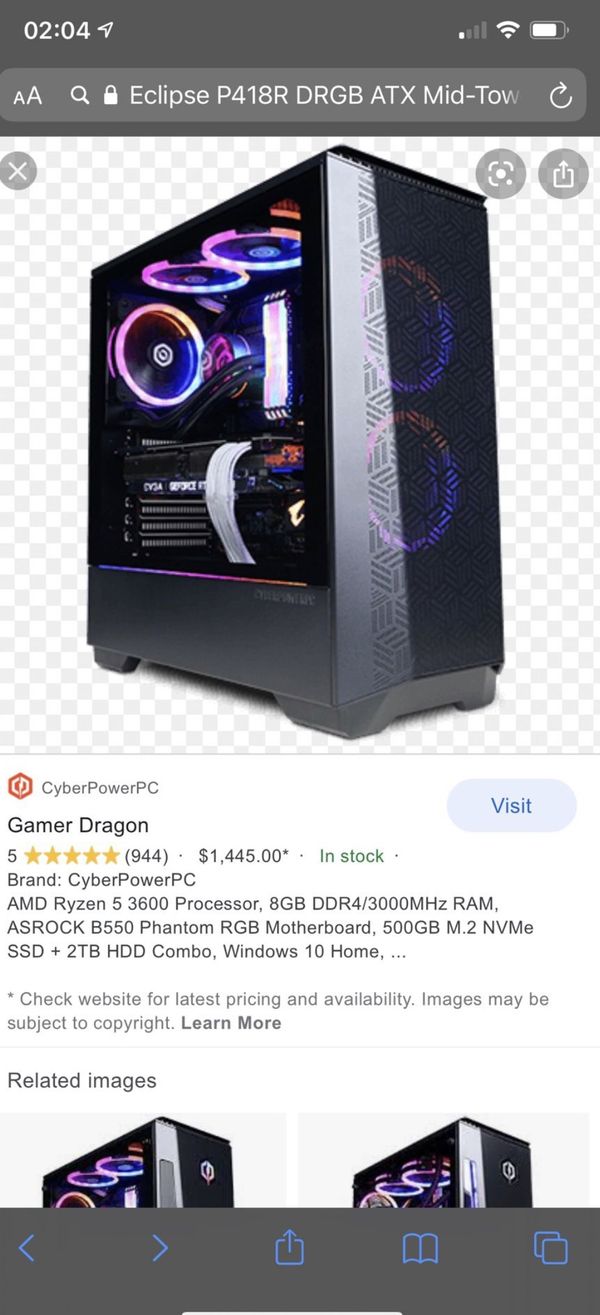The image depicts a smartphone screen displaying various details about a computer tower. At the top of the screen, there's a gray status bar showing indicators such as signal strength bars (4 out of 5), Wi-Fi connectivity, and battery status (mostly charged).

Beneath the status bar, the interface includes a search function with the placeholder text: "Eclipse P 418r dr GB a TX mid - tap to," which appears to be part of the input field.

The main section of the screen features a detailed product description for a "CyberPowerPC Gamer Dragon." The product is highly rated with 5 stars based on 944 reviews, priced at $1,445, and listed as in stock. Key specifications include:
- Brand: CyberPowerPC
- Processor: AMD Ryzen 5 3600
- Memory: 8GB DDR4 RAM (3000MHz)
- Motherboard: ASRock B550 Phantom RGB
- Storage: 500GB M.2 NVMe SSD + 2TB HDD Combo
- Operating System: Windows 10 Home

The description also notes that images may be subject to copyright and advises checking the website for the latest pricing and availability.

The computer tower itself is black with internal lighting in colors such as pink, purple, orange, and yellow, which are visible through its transparent side panel. The website's background or theme also includes these vibrant colors.